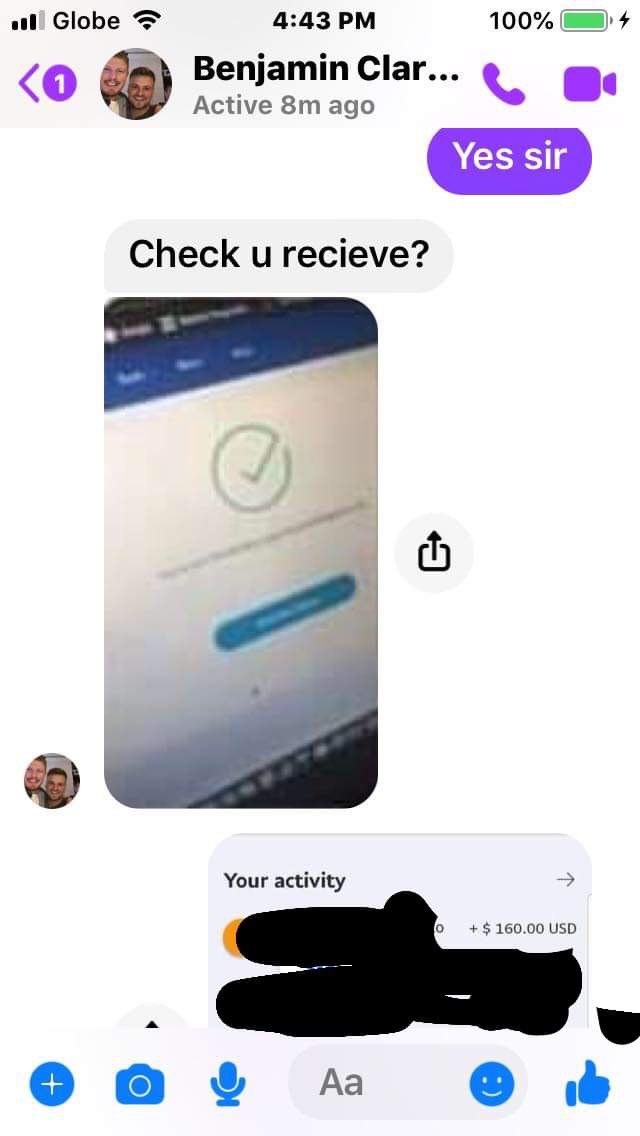This is a detailed screenshot of a conversation on Facebook Messenger, captured on a cell phone. At the very top of the screen, the phone displays full signal strength, Globe as the service provider, and a WiFi connection icon. The battery is fully charged at 100%, and the time is precisely 4:43 PM. The interface shows a light gray header fading to white on the right side.

The conversation is with an individual named Benjamin, whose profile picture, showing two smiling men, is displayed in a circular icon. The context of the messages pertains to a transaction. One message reads "yes sir," adjacent to a blurred screenshot indicating a check mark, followed by the text "check you receive" in another speech bubble. The screenshot appears partially redacted with a section displaying "your activity" and the amount "+160 US dollars" marked out with a magic marker to conceal further details.

At the footer of the chat window, there is an array of Facebook Messenger icons for interaction: a blue circle with a white plus sign, a blue camera, a blue microphone, followed by a text input box with the options "AA" for formatting text, a blue smiley face, and a blue thumbs-up icon for quick responses. 

This detailed setup suggests that the user is actively engaged in a discreet and possibly sensitive transaction with Benjamin, meticulously documenting and discussing a monetary activity.